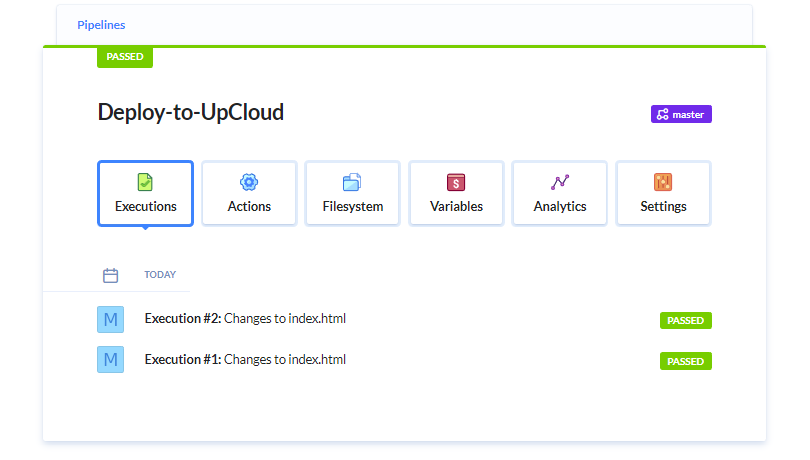The image features a predominantly white background with various elements highlighted in different colors. In the upper left corner, there is a blue text that reads "Pipelines." Directly beneath this, a chartreuse green horizontal line appears, adorned with the word "past" rendered in a white font against the green. Dominating the lower part of the image is the black text "deployed-2-upcloud" in the largest font size.

On the right side of the image, a prominent purple button displays the word "master" in white. Below this button is a vertical list of boxes with labels inside them: "Executions," "Actions," "File Systems," "Variables," "Analytics," and "Settings." The "Executions" box is currently selected, as indicated by a dark blue outline around it, whereas the other boxes have light blue outlines.

Continuing downwards within the "Executions" section, the word "today" is displayed. Just below it, text reads "Execution number two: changes to index.html." Adjacent to this, a chartreuse green button with the word "passed" in white indicates the status. Another entry follows: "Execution number one: changes to index.html," paired with a similar chartreuse green "passed" button.

The overall color scheme includes shades of blue, green, black, white, and purple, suggesting an interface related to software deployment or version control, specifically indicating updates to a website's HTML files.